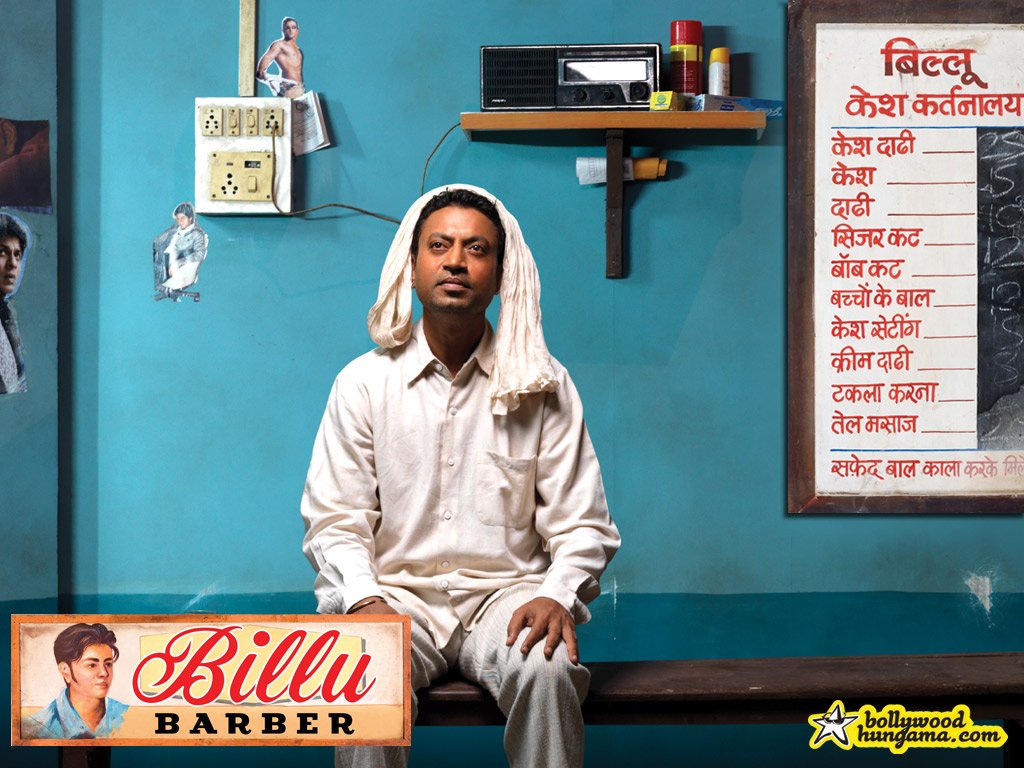The photograph features the renowned Indian actor Irfan Khan seated on a bench at the center of the image, dressed in a white shirt and pants, with a white towel draped over his head. The environment suggests a film still, possibly from "Billu Barber," as indicated by text at the bottom left of the image. He is set against a blue wall that transitions into a darker shade at the bottom, adorned with various elements that add to the scene's richness. An electric panel and plug sockets are visible on the upper left, while the central upper part of the wall features a shelf holding numerous bottles, an old tape recorder, and other miscellaneous items. To the right, a white board displaying text in red Hindi script lists numbers written in chalk. Additional posters and stickers featuring prominent figures can also be seen scattered around the wall. On the bottom right, the logo ‘Bollywood Hungama.com’ is inscribed in black with a yellow border, accompanied by a star icon.